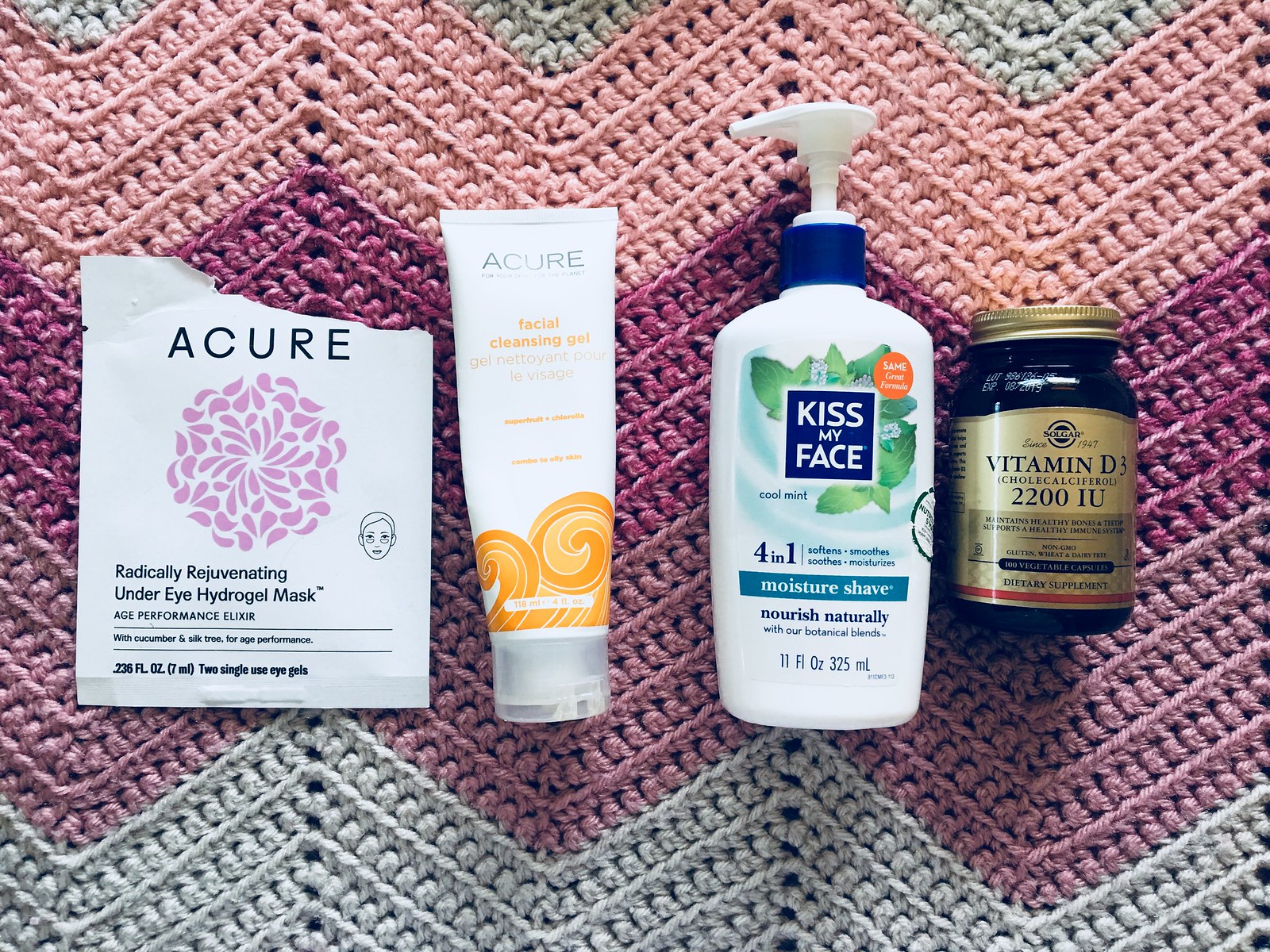The photograph showcases a close-up view of various personal care products displayed on a textured afghan-like material, which features a blend of gray, pink, purple, and pale purple hues. 

1. The first item is a white square package with black font that reads "ACURE". It has an abstract lavender floral motif in the center and is labeled "Radically Rejuvenating Under-Eye Hydrogel Mask" below the design. The packaging also features a small icon of a person's head.

2. The second item is a white tube with a gold-yellow font. It displays "ACURE" in black at the top, followed by "Facial Cleansing Gel" written in the yellow font.

3. The third item is a white pump bottle with a navy, green, and blue design. It prominently reads "KISS MY FACE" in white font on a navy square and is further labeled with "4-IN-1" in navy font and "Moisturize, Shave, Nourish, Naturally" in smaller white font.

4. The final item is a glass bottle with a gold lid and gold label. It has navy font that reads "Vitamin D3 2200 IU" and a distinctive red strip at the bottom of the label.